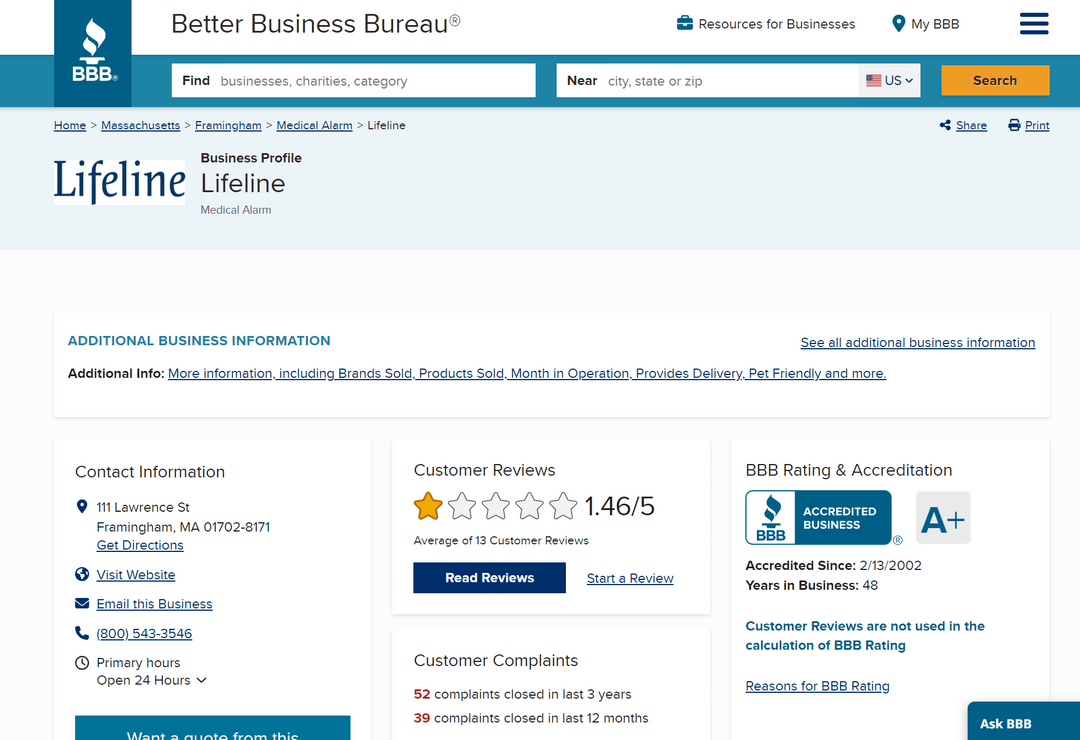This detailed caption presents a clear and structured description of the image:

"The screenshot from the Better Business Bureau website features the profile for Lifeline Medical Admin. Located at 111 Lawrence Street, Framingham, MA 01702-8171, the business provides options for getting directions, visiting their website, and contacting them via email. Additionally, a contact phone number is listed: 800-543-3546. The profile also includes customer feedback, denoted by a rating of 1.46 out of 5 stars."